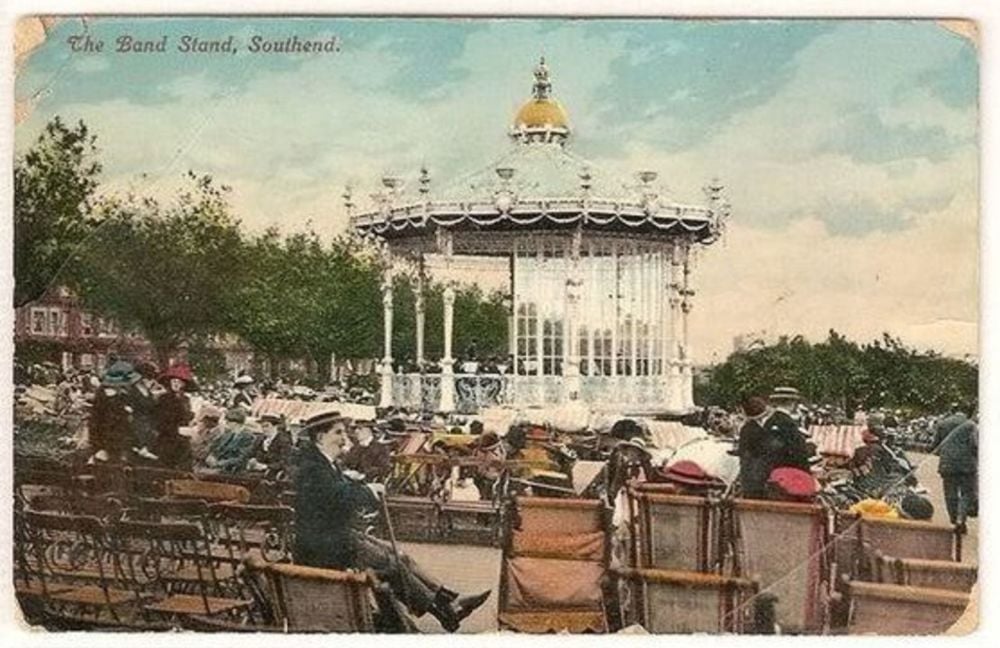The image depicts a vintage scene, possibly from an old postcard or painting, titled "The Bandsand, South End" as indicated by the text at the top. Central to the image is a prominent white bandstand with a striking gold dome, supported by six white pillars. The bandstand appears to be open, with possible band members inside, though their details are indistinct. Surrounding the central structure, the scene extends into what looks like a park adorned with trees and an array of brownish tones, hinting at an old-fashioned or muted color palette.

Numerous chairs are arranged around the bandstand, occupied by people dressed in turn-of-the-century attire. Women in the audience are seen wearing very large hats, long dresses with high collars, and long sleeves, exuding a sense of elegance and propriety. Men are dressed in suits, complemented by straw hats with bands, canes, and black shoes. The overall mood suggests a formal gathering, possibly reminiscent of a carnival or resort atmosphere. The image also reveals minor wear, including small tears at the top left and right corners of the postcard or painting.